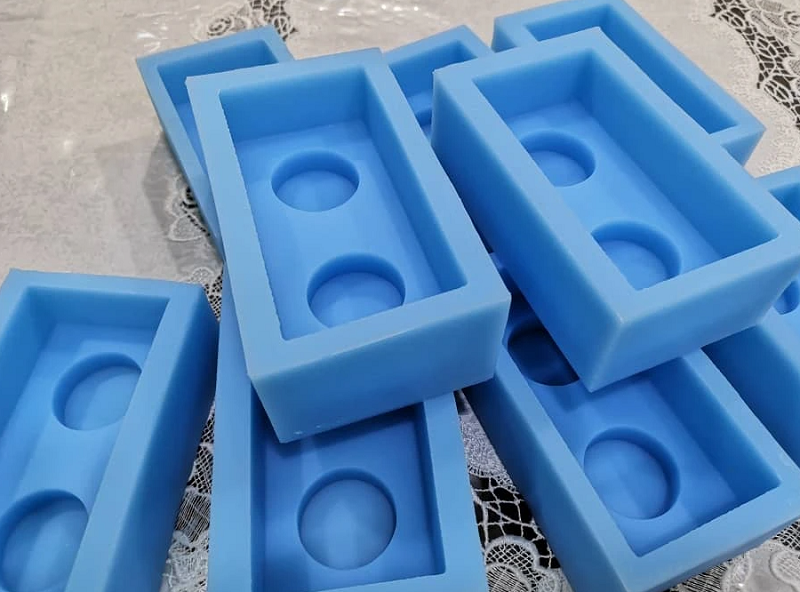The image captures nine light sky blue silicone molds resembling oversized Lego bricks, each featuring two circular connectors. These molds are arranged with two at the top and the remaining seven forming a row of three and a row of four. They rest on a table covered with a white doily, showcasing delicate lace cutouts and floral designs. The lighting casts a fluorescent and reflective glow on the plastic-like surface, enhancing the fine details underneath the molds.